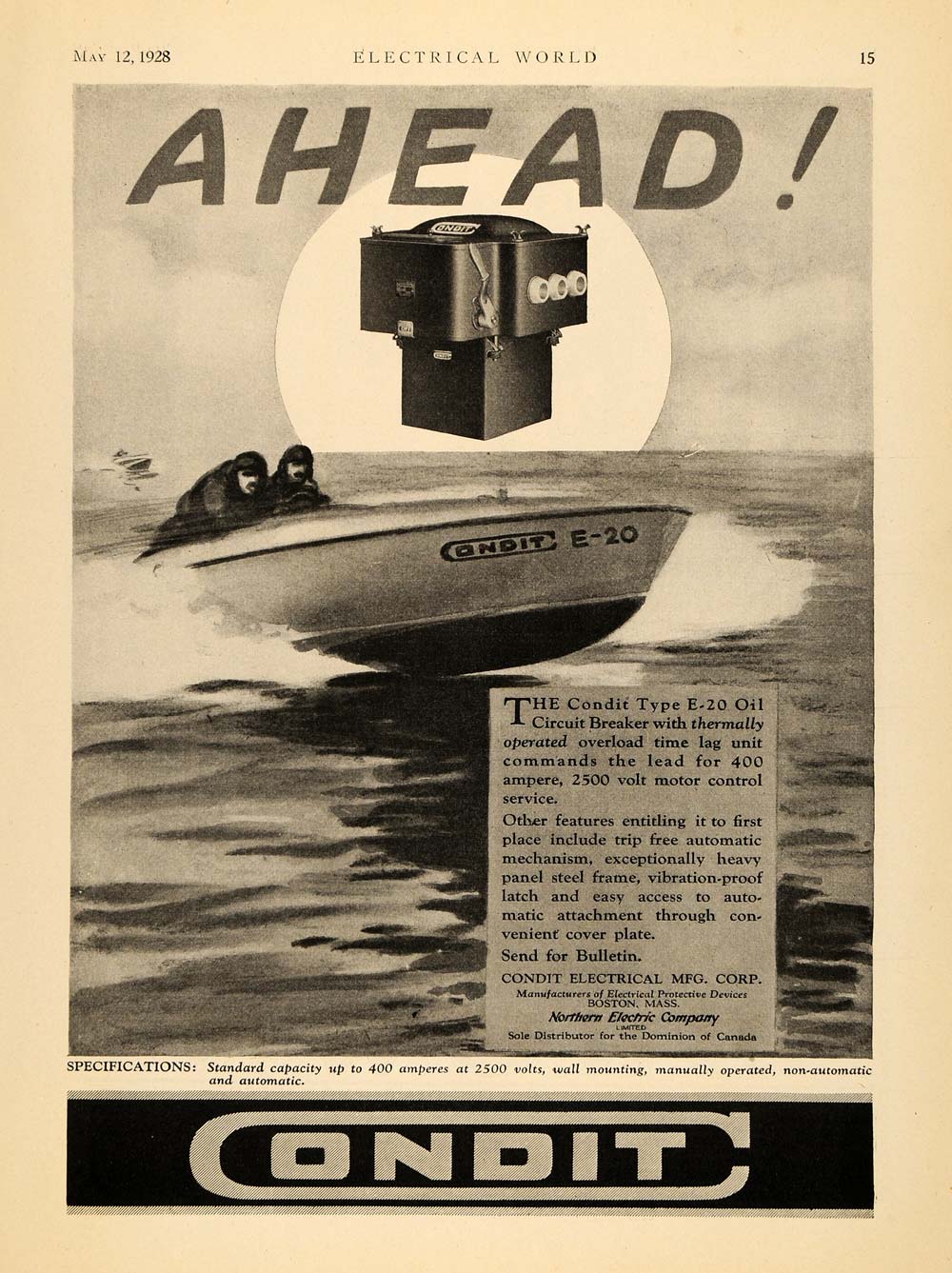This is an advertisement page from the May 12, 1928 issue of Electrical World magazine, specifically page 15. The aged and yellowed page features a black-and-white photograph depicting a speedboat cutting swiftly across the water, with two men clinging to its steering wheel. Behind them, the sun is low on the horizon, suggesting a sunset scene. Prominently displayed above the boat is the word "Ahead!" Below the boat, a detailed description extols the virtues of the product being advertised: the Condon Type E20 Oil Circuit Breaker with Thermally Operated Overload Time Lag Unit. It highlights its lead in 400 amp, 250 volt motor control service, mentioning features such as a trip-free automatic mechanism, heavy panel, steel frame, vibration-proof latch, and easy access through a convenient cover plate. A recognizable black banner at the bottom of the page carries the company's name, "Condon," stylized with an oval pattern encircling the letters "O-N-D-I-T."